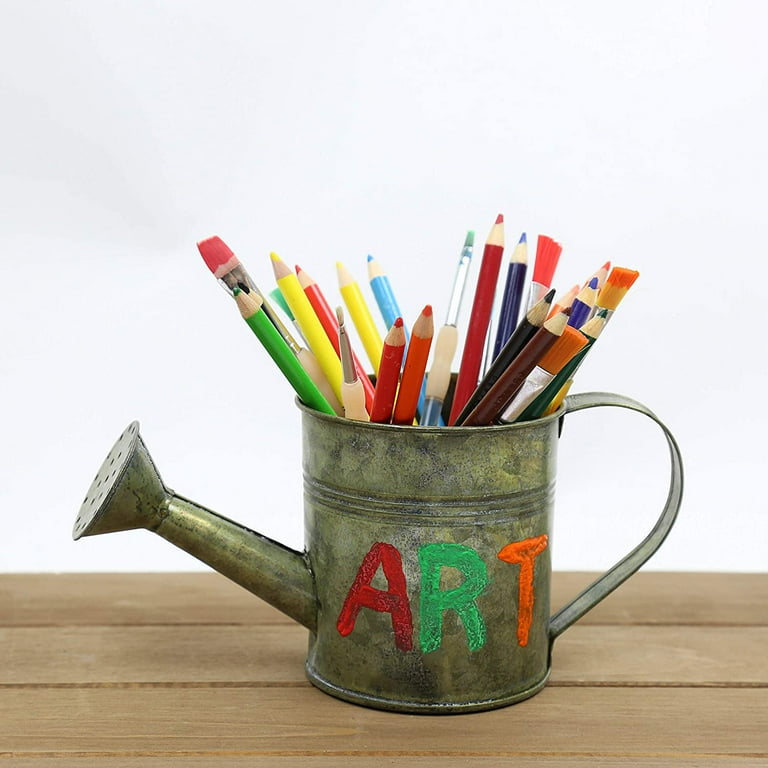The photograph depicts an old, discolored metal watering can, likely made of brass, characterized by a green and olive patina from age. It features a perforated spout designed for a gentle spray, typical of such gardening tools. On the front of the can, the word "ART" is painted in childlike, simple capital letters: the A in red, the R in green, and the T in orange. Above the word "ART," there are three indentations encircling the cylindrical part of the can. The curved handle arches on the right side of the watering can. The can, repurposed as a holder, contains various art supplies including colored pencils—yellow, red, blue, light green, black, beige, teal, orange, purple, and brown—as well as several paintbrushes with red, orange, and green-tipped bristles. The weathered and artistic watering can sits on a wooden table against a plain, white background, evoking a sense of creativity and nostalgia.